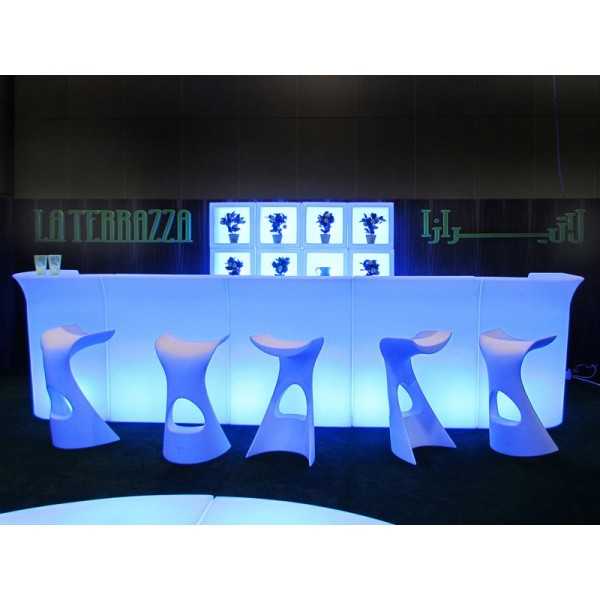This image depicts a graphically designed nightclub bar with a distinctive modern aesthetic. The bar itself emits a purple glow from its opaque structure, suggesting a type of glass enclosure with internal lighting. The seating consists of five uniquely curved stools without backs, adding an improbable, contemporary flair. Behind the bar, shelves adorned with plants are backlit with white light, providing a striking contrast against the dark walls and ceiling. On the wall, the name "La Terraza" is prominently displayed alongside additional text in Arabic characters. At the end of the bar, two glasses are poised, adding a final touch to this sophisticated and eclectic scene.